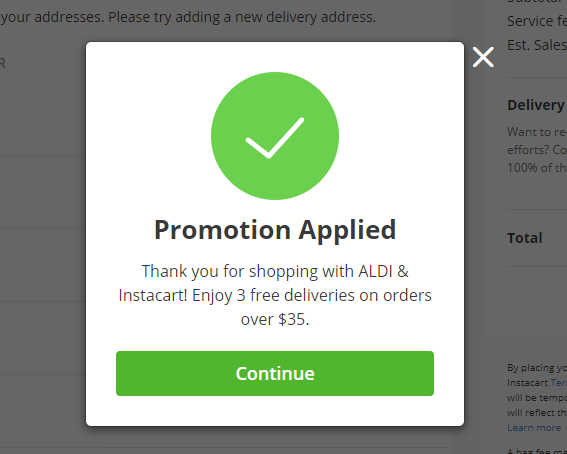The image features a dark gray background with a prominent white box centered in the middle. On the upper right corner of this white box is a white "X" indicating a close button. Within the box, a large green circle occupies the center, emblazoned with a white checkmark, symbolizing success. Below this circle, the text reads: "Promotion Applied. Thank you for shopping with Aldi and Instacart. Enjoy three free deliveries on orders over $35."

Towards the bottom of the white box, there is a large green button labeled "Continue." The gray background around the box displays various sections related to delivery options, total amount, and fields for order details. Near the top of the image, there is information pertaining to addresses with a prompt suggesting the addition of a new delivery address. 

In essence, this announcement confirms that the promotion has been successfully applied and encourages the user to proceed by clicking the "Continue" button, while details of the order and additional options frame the main message.